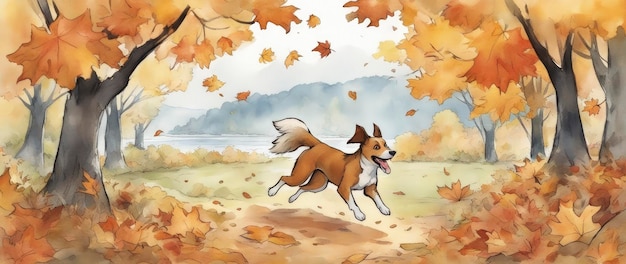This detailed illustration depicts a joyful brown dog with white patches on its neck, belly, chest, paws, and the tip of its tail, prancing energetically to the right in an autumnal woodland clearing. The dog’s ears are blown back by the wind and its tongue hangs happily out of its mouth. The background reveals a serene body of water bordered by a dense wood line of leafy trees, with additional hills covered in foliage. The scene captures the essence of fall with large maple leaves in vibrant orange and yellow hues drifting to the ground and forming big piles under the trees. The overall atmosphere suggests a foggy fall day, enhancing the feeling of the season as the dog enjoys its playful romp in the meadow, unaccompanied by other animals and text.